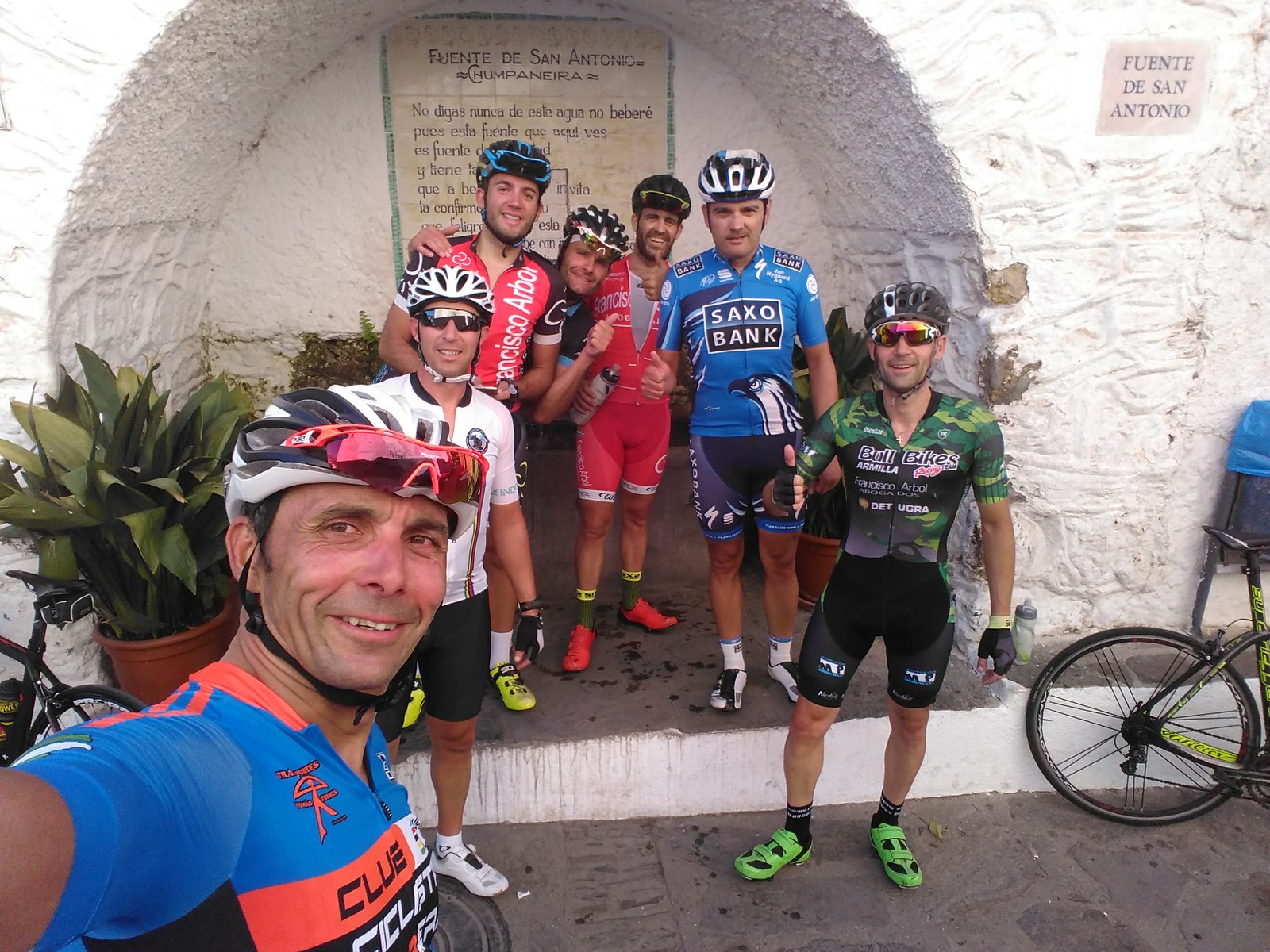In this vibrant and energetic photo, a group of enthusiastic male cyclists, likely in their 30s, are gathered together, posing for a selfie taken by the frontmost rider. He is identifiable by his blue and orange shirt, contrasting with the array of colorful biking outfits adorned with sponsorship logos that the other riders wear. All seven men are equipped with helmets, and they display a joyful camaraderie, with some giving thumbs up.

They are positioned in front of an arch made of white stone, with a distinct plaque that reads, "Fuente de San Antonio," suggesting a picturesque location, possibly in Italy or Spain. The setting includes a large shrub behind the central figure and a stone building with an inscription. Four of the cyclists are standing under the arch, while the remaining three are positioned on the ground level. Bicycles can be seen parked to the side, enhancing the aura of a well-organized cycling adventure.